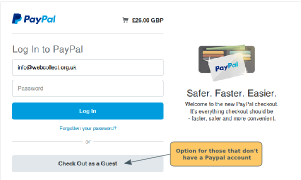The image depicts a PayPal login screen. In the top left corner, the PayPal logo is prominently displayed. To the right of the logo, there's a small shopping cart icon with the text "26 GBP" (GBP indicates British Pounds). A vertical separating line follows, leading to the "Log In to PayPal" section.

This section contains two input boxes: the first one, which is unreadable, presumably for a username or email address, and the second for the password, labeled "Password" but currently blank. Below these boxes is a blue "Log In" button. Further down, there's a link with the text "Forgot your password?"

Another horizontal separating line is present with the word "or" in the middle. Below this, there's the option to "Check Out as Guest," indicated by an arrow originating from a yellow speech bubble. This bubble contains the text "Option for those who don't have a PayPal account."

At the top of the screen, an image shows a PayPal card and a wallet with the slogan "Safer, faster, easier." Some additional, blurry text is present, which is difficult to read.